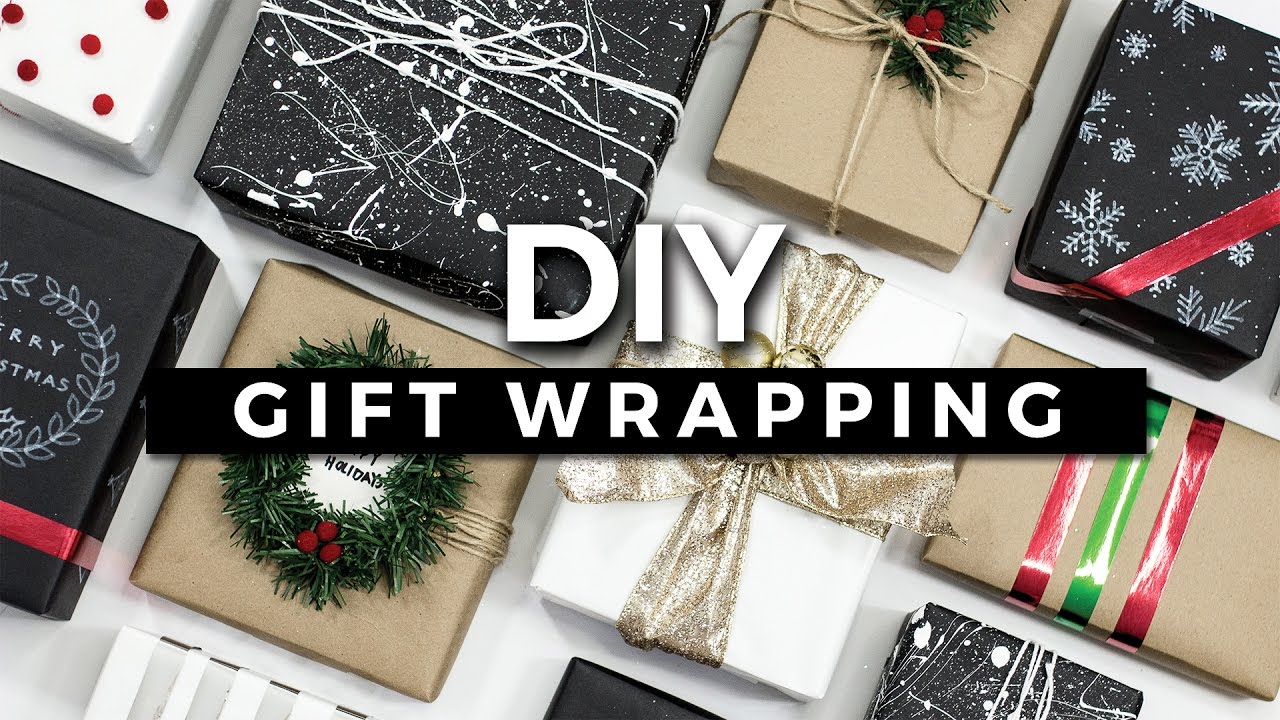The horizontal rectangular image appears to be a screenshot or a graphic for digital content such as a website banner or a YouTube video. The focal point of the image is the bold, all-caps white text "DIY" prominently displayed across the center. Directly beneath this, a horizontal black stripe spans the width of the image, featuring spaced-apart, all-caps white text that reads "GIFT WRAPPING."

The background showcases a festive assortment of wrapped presents spread across a white countertop. These presents are meticulously wrapped in a variety of colors and patterns, creating an eye-catching display. The gift wrap styles range from minimalist, earthy brown paper tied with brown twine, to more elaborate designs including red and green ribbons, gold bows, and green Christmas wreaths. Some presents are adorned with black paper splashed with white paint, others with all-white paper dotted with golden stars or red dots, and some feature black paper with white snowflakes. The overall theme exudes a Christmas vibe, highlighted by the frequent use of traditional holiday colors and motifs. This image effectively captures the spirit of holiday gift-giving and the art of creative DIY gift wrapping, making it an appealing visual for seasonal content.